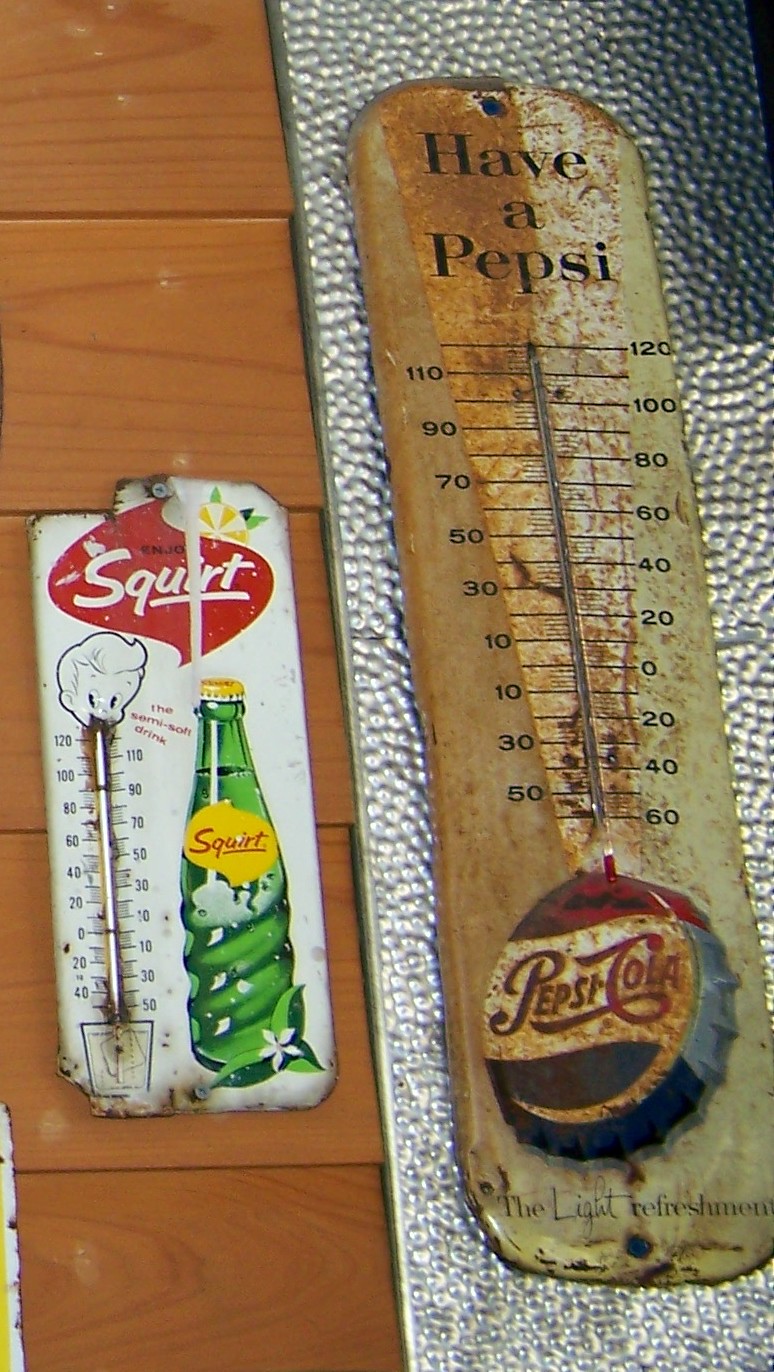The photograph captures two vintage advertising thermometers hanging on a wall made of horizontally paneled real maple wood. 

The thermometer on the left is an advertisement for Squirt, a lemon-lime flavored soft drink. This nostalgic piece features a cartoon image of a young individual sipping through the thermometer's mercury tube, which appears to be dipped into a glass at the bottom. A classic 10-ounce Squirt bottle is displayed on the right side of this illustration with the Squirt logo prominently at the top. The thermometer is affixed to the wall with screws, and some parts are missing due to age.

On the right side of the image is a significantly larger Pepsi thermometer, which harkens back to a time when such items would have adorned the outer walls of old-fashioned general stores. The Pepsi thermometer is visibly weathered and soiled, adding to its vintage charm. It is mounted against a textured, silver metal surface. At the bottom, it carries the slogan "The Light Refreshment" along with a call to action, "Have a Pepsi."

Together, these vintage thermometers encapsulate a rich history of mid-20th-century advertising aesthetics.